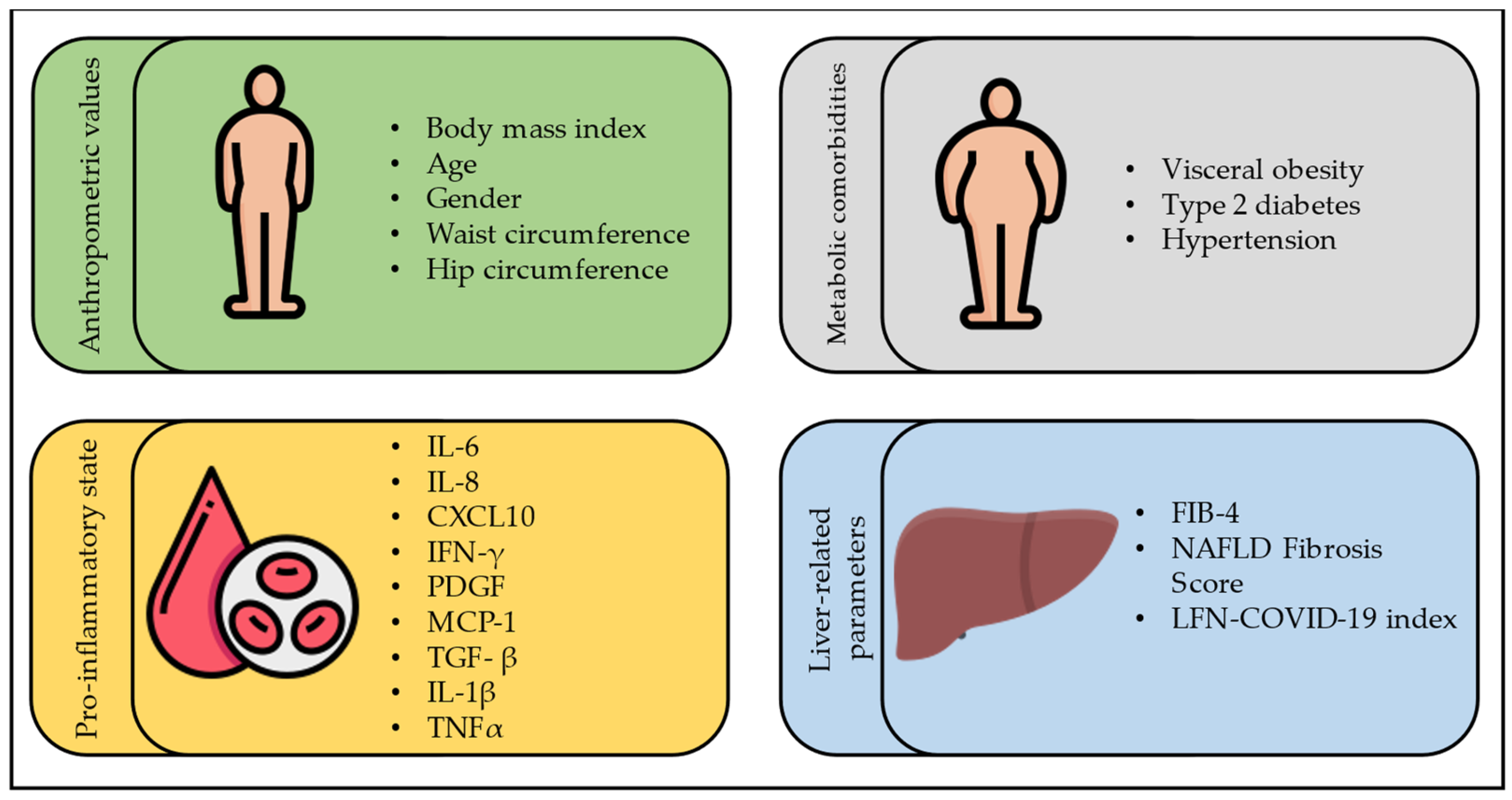The image features a detailed, diagrammatic page with four rounded, horizontally-oriented rectangles, each dedicated to specific health-related topics. 

In the upper left, within a green rectangle labeled "Anthropometric Values," lies a simplistic human figure, marked with key health metrics: body mass index, age, gender, waist circumference, and hip circumference.

To its right, encased in a gray rectangle labeled "Metabolic Comorbidities," is a larger outlined human figure. This section highlights conditions such as visceral obesity, type 2 diabetes, and hypertension.

The lower left features a yellow rectangle, labeled with "Pro-Inflammatory State," illustrated by a red teardrop and a white circle containing red dots. This section lists various inflammatory markers: IL-6, IL-8, CXCL-10, IFN-Y, PDGF, MCP-1, TGF-B, IL-1B, and TNFA.

To the right, in a blue rectangle titled "Liver-Related Parameters," there's an illustration of a liver. It includes metrics like FIB-4 and NAFLD fibrosis score, as well as an LFN-COVID-19 index.